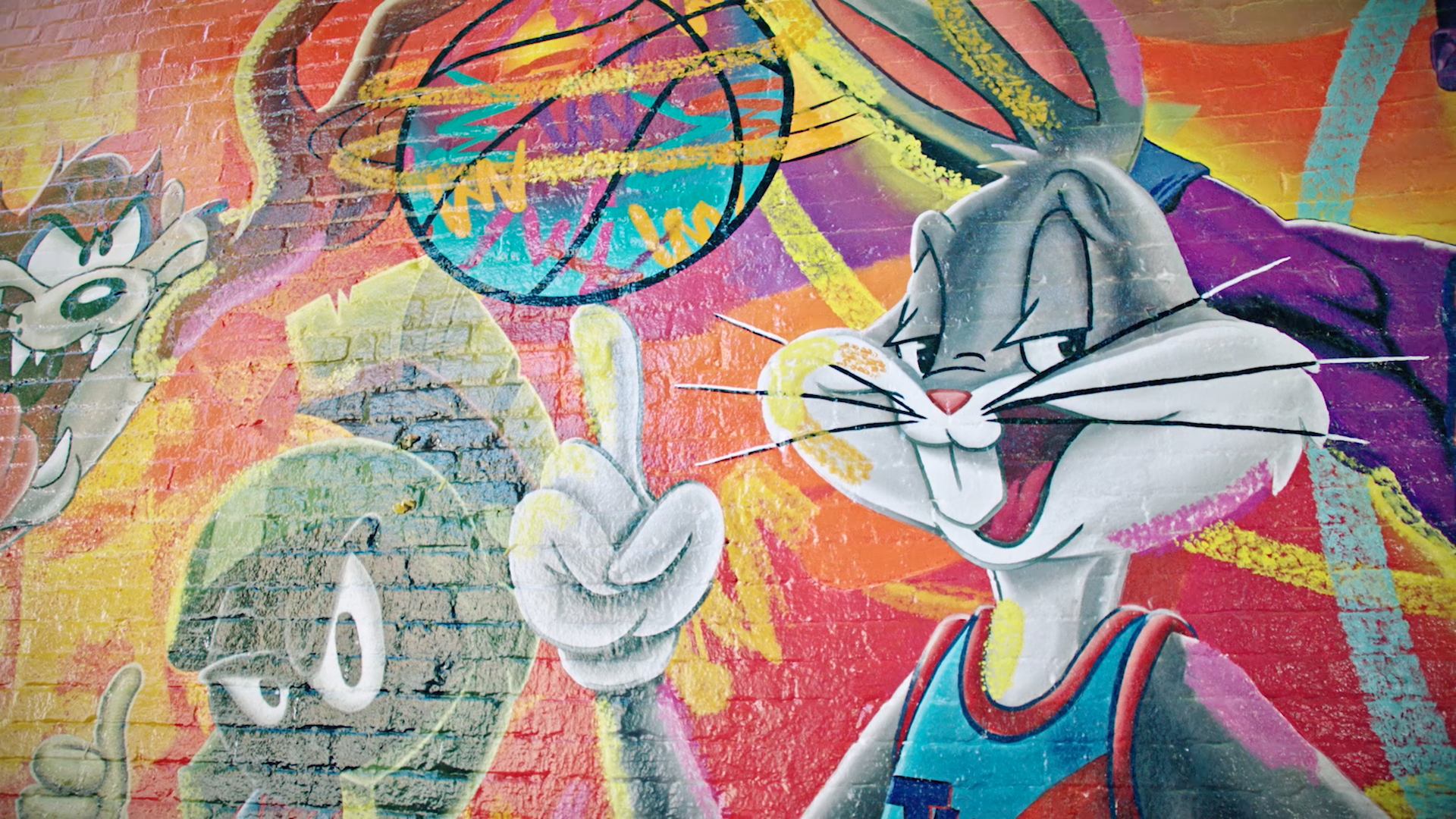The outdoor mural on a brick wall features vibrant depictions of three iconic Looney Tunes characters. Dominating the right side, Bugs Bunny, dressed in a basketball uniform, twirls a colorful, multicolored basketball on one of his gloved fingers while looking directly at the viewer, his mouth open as if talking. To his left stands Marvin the Martian, distinguishable by his green helmet with a matching mohawk and his black face, giving a thumbs-up sign and raising an eyebrow in a manner reminiscent of Dwayne Johnson. Lastly, on the far left, the Tasmanian Devil, Taz, appears to be lunging and reaching for Bugs Bunny's basketball, with his typical wild expression, fangs bared, and tongue hanging out. The mural is set against a background filled with abstract splashes of yellow, red, purple, and blue stripes, adding to the dynamic and colorful scene.